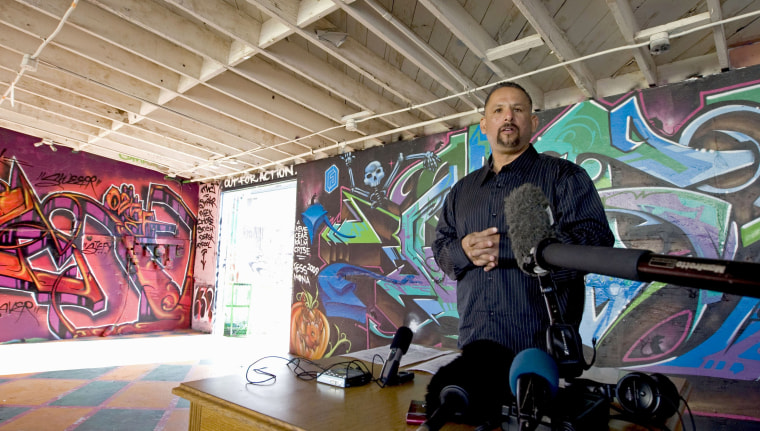In the photograph, a man in his 40s, possibly Latino, stands behind a large, light brown desk covered with various audio equipment. He is wearing a vertically striped button-down shirt with dark blue and light blue colors. The man, who has a goatee and short hair, appears to be speaking, possibly in a classroom or studio setting. The desk is cluttered with black microphones, a microphone on a stand with a fluffy cover, black headphones, a black speaker, and a few white papers.

The room around him is vibrantly decorated with graffiti artwork featuring a range of colors including purple, blue, green, pink, and red. One wall displays a detailed skeleton painting. The graffiti designs have a cyberpunk aesthetic, with various shapes and letters. There's an additional orange pumpkin painted in a corner. The ceiling is wooden with painted white joists, adding a rustic touch to the otherwise urban art-filled space. The floor has a checkered pattern in black, pink, and orange, which could be tile or linoleum. An open doorway allows light to stream into the room, suggesting it's daytime outside. Overall, the scene is dynamic and visually stimulating, blending the artistic interior with the functional audio setup.